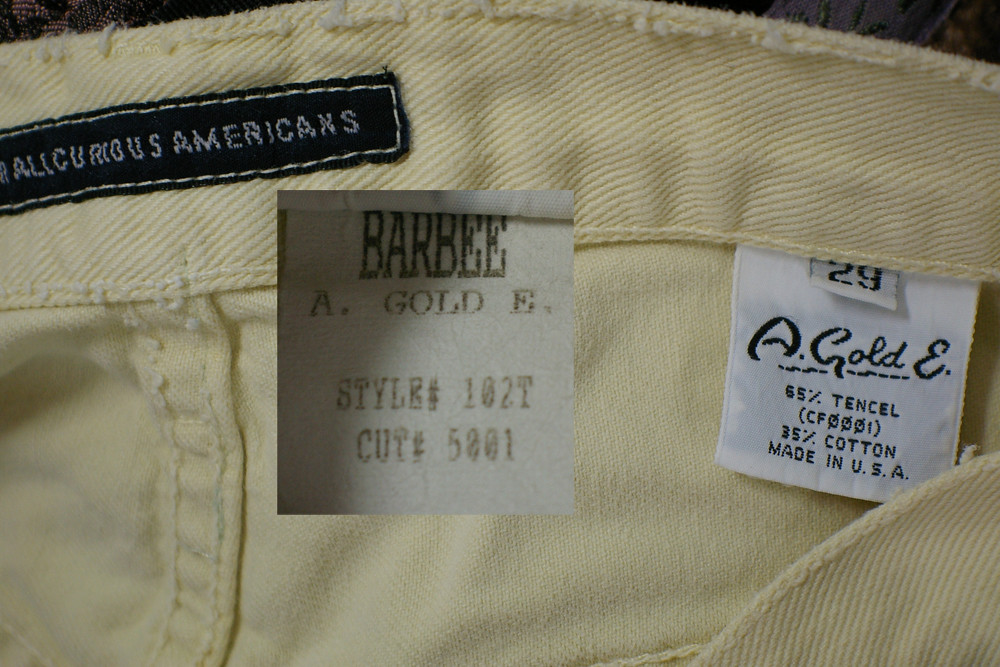In this detailed close-up photograph, we see the interior of a pair of pants made by the brand "All Curious Americans," featuring a creamy, light-yellow, denim-like material that is durable and well-constructed. The primary focus of the image is on three distinct tags. In the top left-hand corner, a black label states "All Curious Americans." Below it, on the lower right side, a tag reads "Barbie, A. Gold E., Style 102 T, Cut 5201," and appears slightly out of place. On the right side, another standard white tag displays "2-9, A. Gold E., 65% Tencel, 35% Cotton, Made in the USA," indicating the materials and manufacturing details. The fabric near the waistband appears to be frayed, suggesting either wear or a designer's intentional distressed style. This garment, presumed to be pants, has a high-quality look and maintains a distinct, stylish appearance highlighted by its unique tagging and light banana hue.